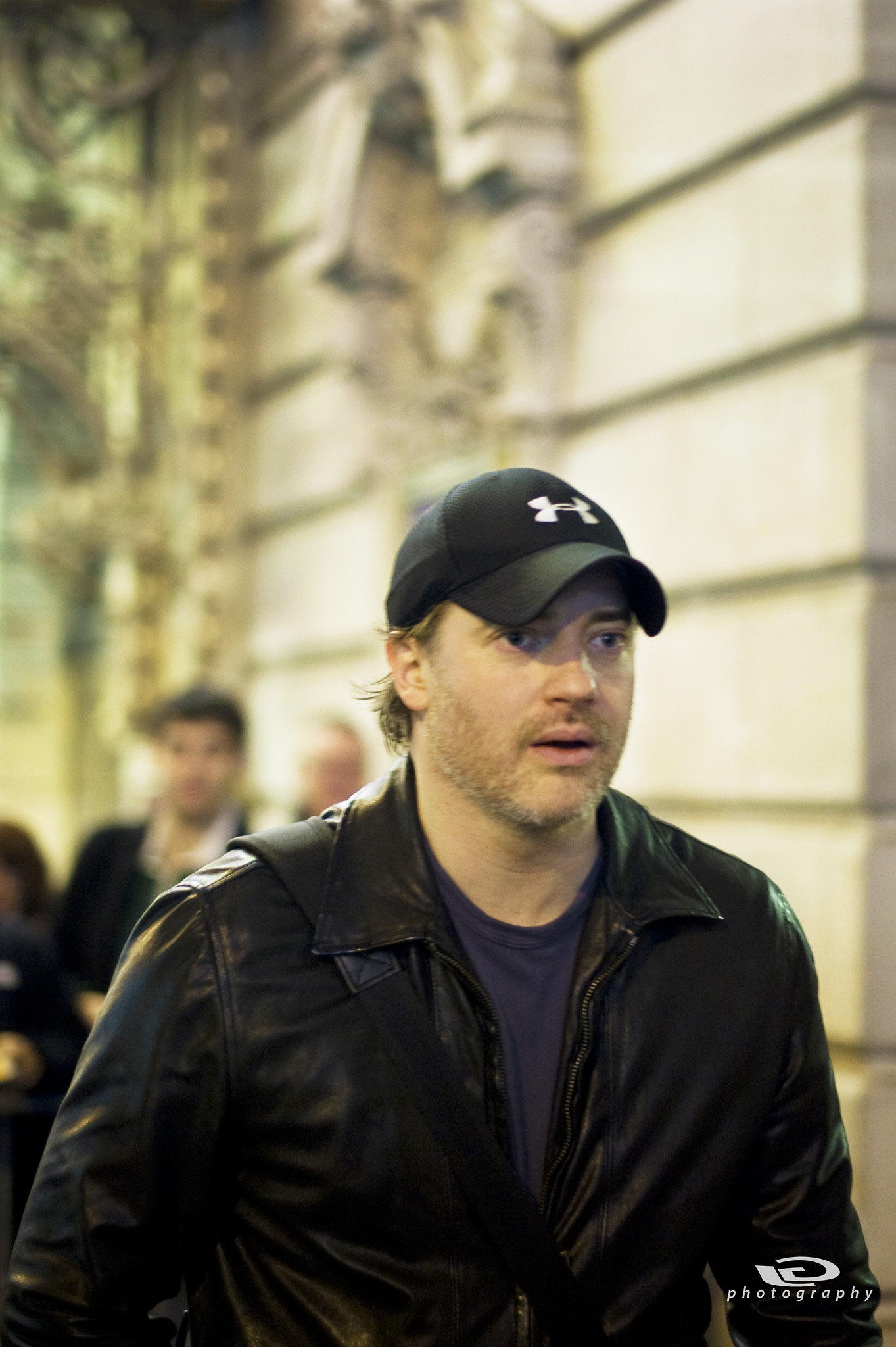The image features actor Brendan Fraser walking down the street in casual attire. He is wearing a black leather jacket over a blue t-shirt, with a black crossbody bag strap visible over his shoulder. He has light brown facial hair with hints of gray, and he dons a black Under Armour baseball cap with a white "H" logo. Fraser appears to be deep in thought, looking slightly to the right, with his mouth partly open. Behind him, there are several blurred figures, including a man in a suit, against the backdrop of a tall building with a white, possibly limestone, facade featuring lateral lines. The photo is brightly lit, and in the bottom-right corner, there's a partially legible white logo that includes the word "photography."